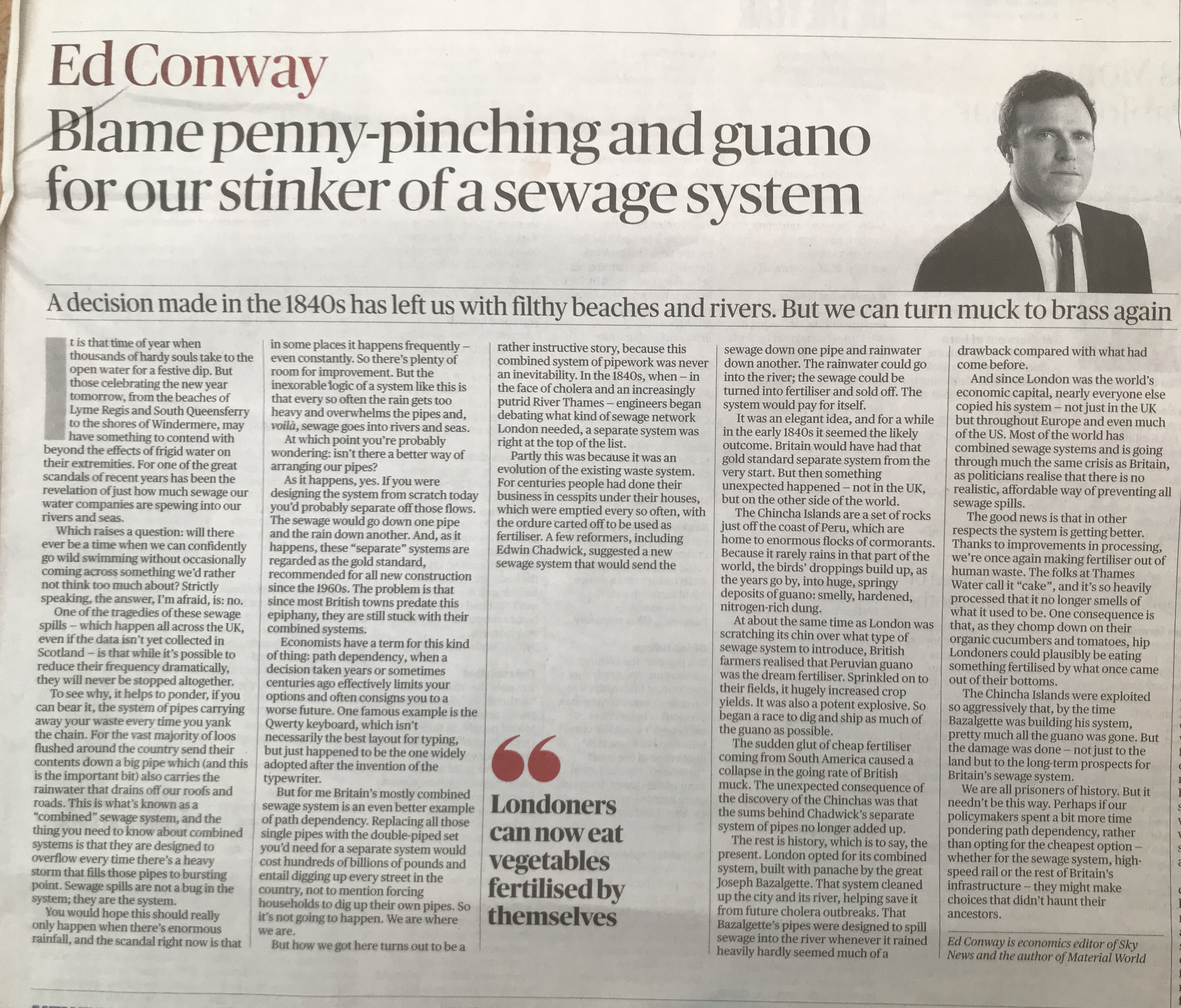This image is a JPEG photograph, likely intended for online display. It showcases a physical newspaper page with noticeable details such as crinkled paper in the upper left corner and an overall tilt to the right, indicating it wasn't squared up properly. The headline is prominently printed in a burgundy-red ink, stating "Ed Conway," and beneath it in black ink, "Blame Penny Pinching and Guano for Our Stinker of a Sewage System." Accompanying the article is a black-and-white photo of a man in a black suit and white shirt, identified by his short brown hair. The subheadline mentions that a decision made in the 1840s has resulted in polluted beaches and rivers, but suggests there is potential to turn this situation around. The article spans five columns, with the middle column cutting off midway. Above a related quote, in large red symbols, it says, "Londoners can now eat vegetables fertilized by themselves," in heavy black text. The byline at the bottom identifies Ed Conway as the economics editor of Sky News and author of "Material World," confirming that this page is from a Sky News publication.